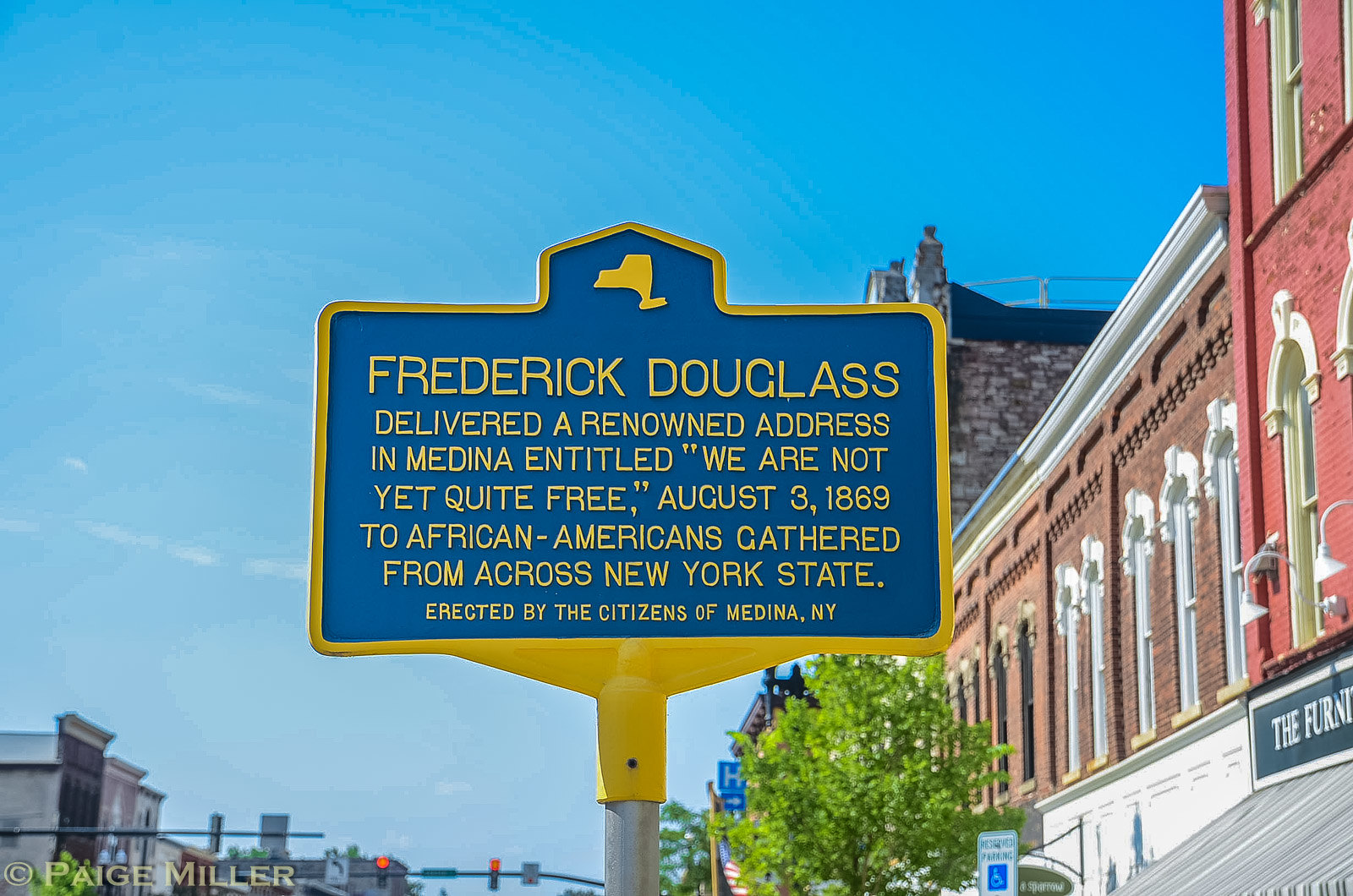This photograph captures a well-maintained historical sign prominently displayed in the downtown area of Medina, New York. The sign, framed with a yellow outline and featuring a yellow silhouette of New York State on a blue background, commemorates an address delivered by Frederick Douglass on August 3rd, 1869, titled "We Are Not Yet Quite Free." This notable speech was given to a gathering of African Americans from across New York State and the sign was erected by the citizens of Medina, New York. The surroundings of the sign include vintage brick buildings on both sides, trees, and handicap parking signs, suggesting an old-town atmosphere. In the background, red stoplights and a clear blue sky with few, if any, clouds are visible, emphasizing the sign as the main focal point.